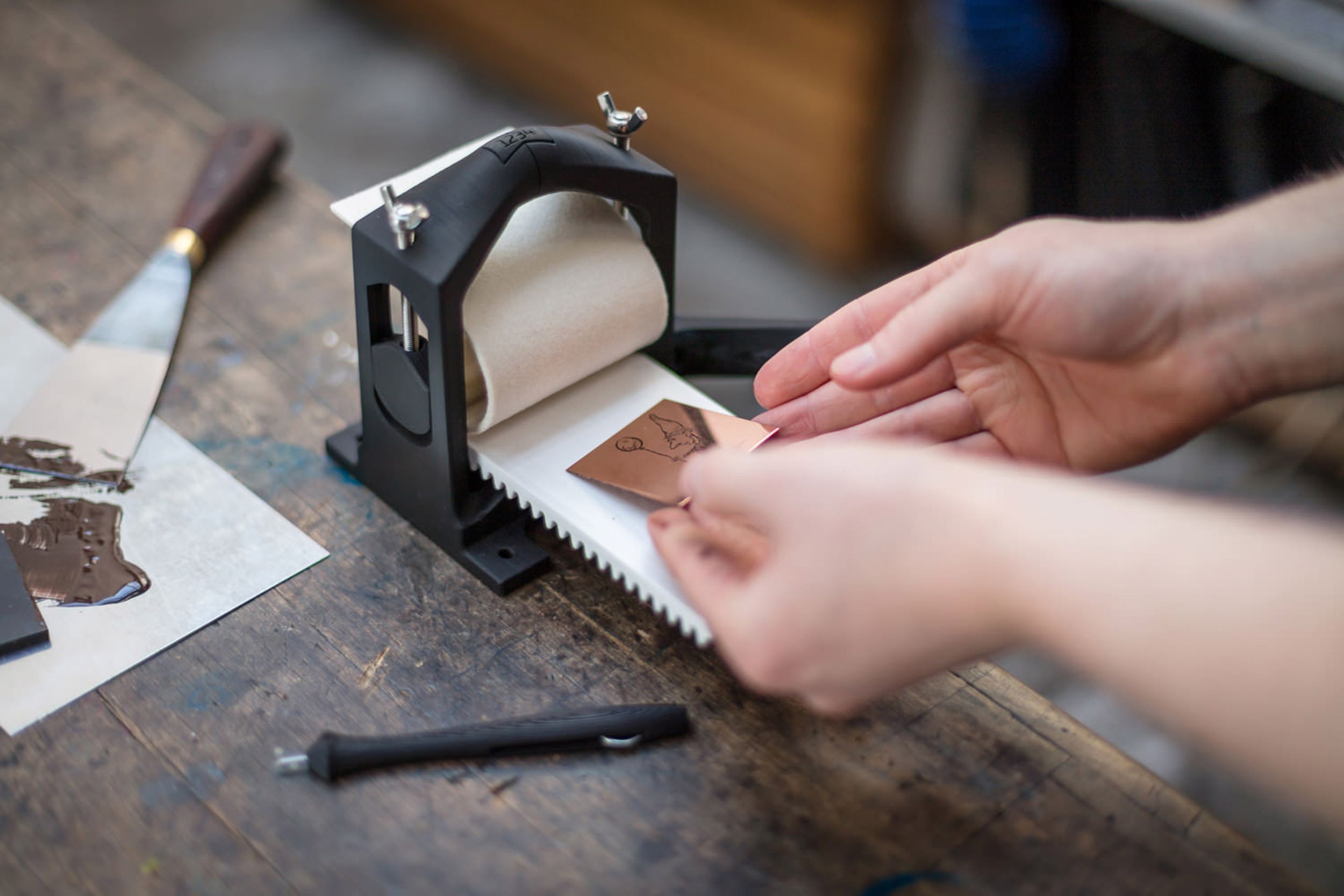The image captures a detailed scene of a person engaged in a meticulous process at a workshop. The focal point is a small, black, metal contraption, likely a miniature printing press, clamped to the edge of an old, heavy wooden table. Two hands, appearing from the right, hold a small copper or brass plate with an intricate etching that resembles a wizard holding a balloon. The person is carefully positioning this plate onto a roll of thin paper or cloth secured in the press. To the left of the press lies a black, pen-shaped instrument and a spatula or putty knife beside some greaseproof paper with what appears to be brown ink or putty. The surrounding table area is intentionally blurred, drawing attention to the central action of the plate being aligned for a possible printing or pressing process.